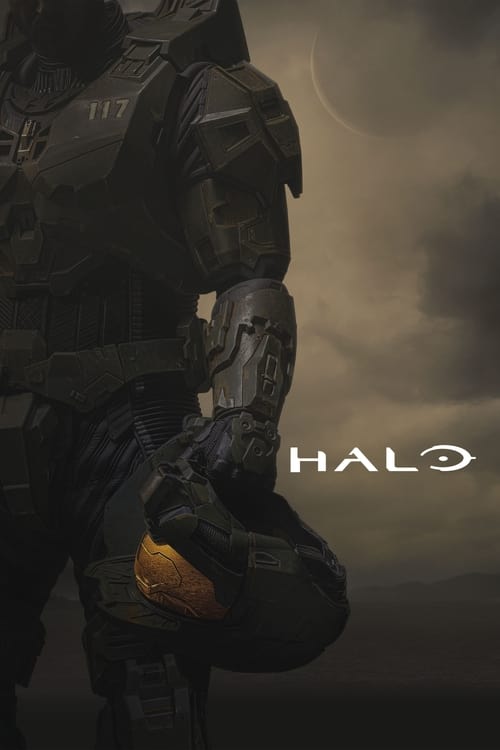The image is a promotional poster for the Halo franchise, showcasing the iconic character Master Chief. Dominating the left side of the image, Master Chief is seen from the neck down, clad in his recognizable black or dark gray armor which is marked with the number 117 on the right chest plate. His heavily armored figure is partially cut off at the ankles, giving a sense of his towering presence. He holds his helmet by his side in his jointed, armored hand. The helmet, matching the dark armor, features a reflective visor. The background presents a moody, stormy sky with dark gray clouds and a partially visible crescent moon in the upper right corner, adding a dramatic atmosphere. On the right side of the image, in bold white font, the word “HALO” is prominently displayed, underscoring the image's connection to the renowned video game series and its adaptation into the Paramount Plus television series. The overall tone is dark and foreboding, reflecting the intense and epic nature of the Halo universe.